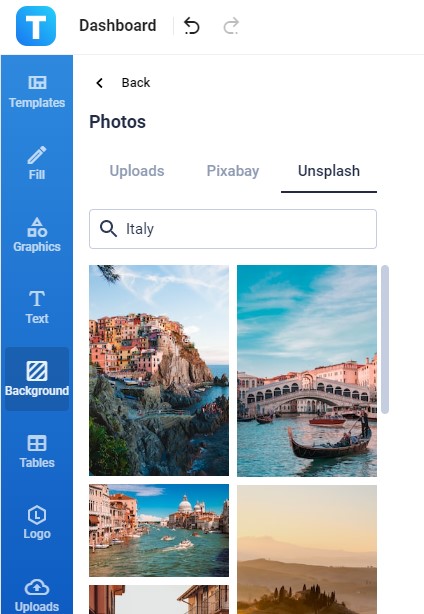This image is a screenshot from a photo editing software or app interface. In the upper left corner, there is a white uppercase "T" encased in a blue rectangle. To the right of this icon, in black font, it says "Dashboard." Above this text are navigation arrows: a curved left-pointing arrow for the back button and a similar arrow pointing right, which is grayed out indicating it is currently inactive.

On the left side of the interface, there is a vertical blue rectangle featuring several white-labeled editing options: Templates, Fill, Graphics, Text, Background, Tables, Logo, and Uploads. The "Background" option is currently selected, indicated by a slightly darker blue shade and bolder white text.

At the top of the interface, there is a horizontal menu with "Unsplash" highlighted in bold black font and underlined, signaling it is the active selection. To the left of "Unsplash," options for "Pixel Bay" and "Uploads" are also present. Directly beneath this menu, a search bar is visible with the query "Italy."

Displayed below the search bar are multiple images depicting various Italian landscapes, featuring water, cities, and natural areas of Italy. These photos are part of the search results provided for the term "Italy."